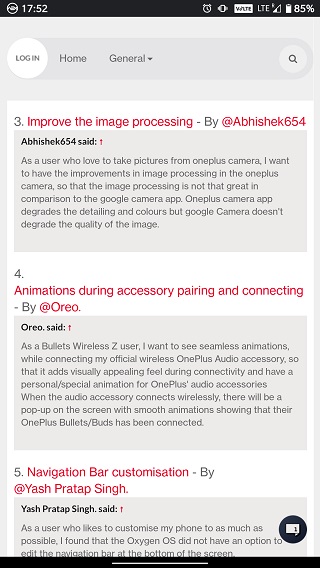The image depicts a smartphone screen showing a community message board interface at 17:52, with various user posts about software improvements. In the top-left corner, there is a time display '17:52', and on the top-right corner, there are standard phone icons including battery charge. Below the time, a white circle with 'Login' is visible on the left.

Across the top, navigation options include 'Home' and 'General,' with 'General' sporting a downwards arrow. On the right side of this bar, there is a magnifying glass icon indicating a search function.

The main content area displays user posts:
1. The top post is highlighted with a red label 'Improve the image processing,' listed as number 3 and authored by 'Abhishek654.' The post reads, "As a user who loves to take pictures from OnePlus camera, I want improvements in image processing. Currently, the detailing and colors are degraded compared to the Google camera app, which maintains the quality of the image." This text is in a grey box.
2. The next post, by '@Oreo,' is titled 'Animations during accessory pairing and connecting.' Below the title, there is a paragraph discussing the topic.
3. The final post, titled 'Navigation bar customization,' is authored by '@Yash Pratap Singh' and also includes a paragraph elaborating on the user's suggestion.

The image captures user feedback and suggestions aimed at enhancing the functionality and user experience of the OnePlus camera and related features.